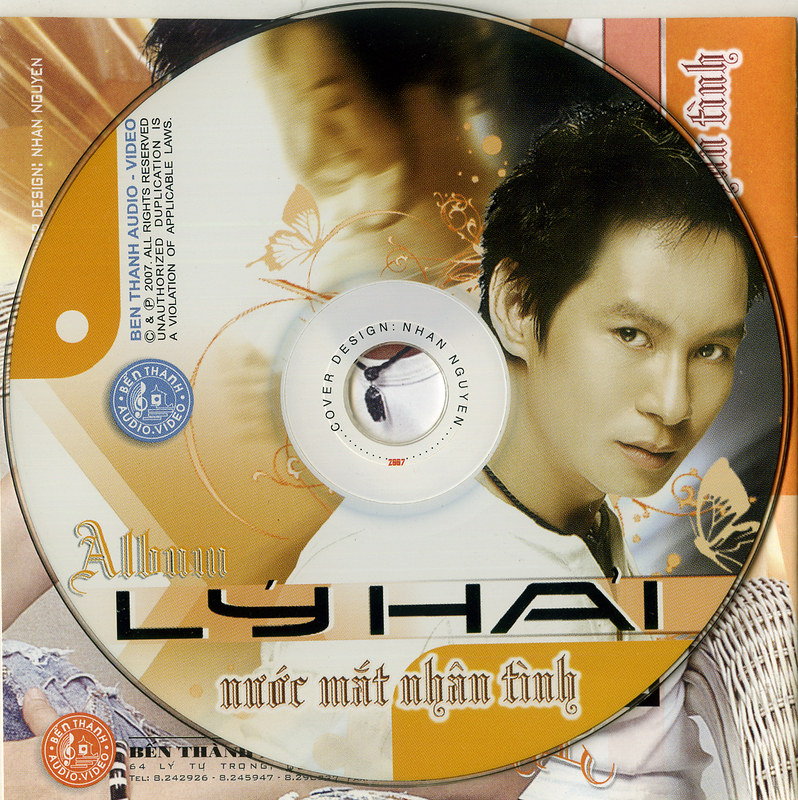This full-color image depicts a CD with an orange and white color scheme. Dominating the right side of the CD is a photograph of a young Asian male with short black hair, a serious gaze, and a few strands of hair starting to cover his forehead. He is dressed in a white shirt and a black braided necklace. The man's name, "L Y H A I," is prominently displayed below his image in black text, along with additional text in Vietnamese, indicating that he is a Vietnamese recording artist. The background includes a blurred image of a dark-haired female with her hair tied up, adding depth to the design. Notable design elements include butterflies printed on the CD—one to the bottom right of the male's face and another above his ear. The CD design is credited to Nahon Nguyen, emphasizing the artistic effort put into the cover.